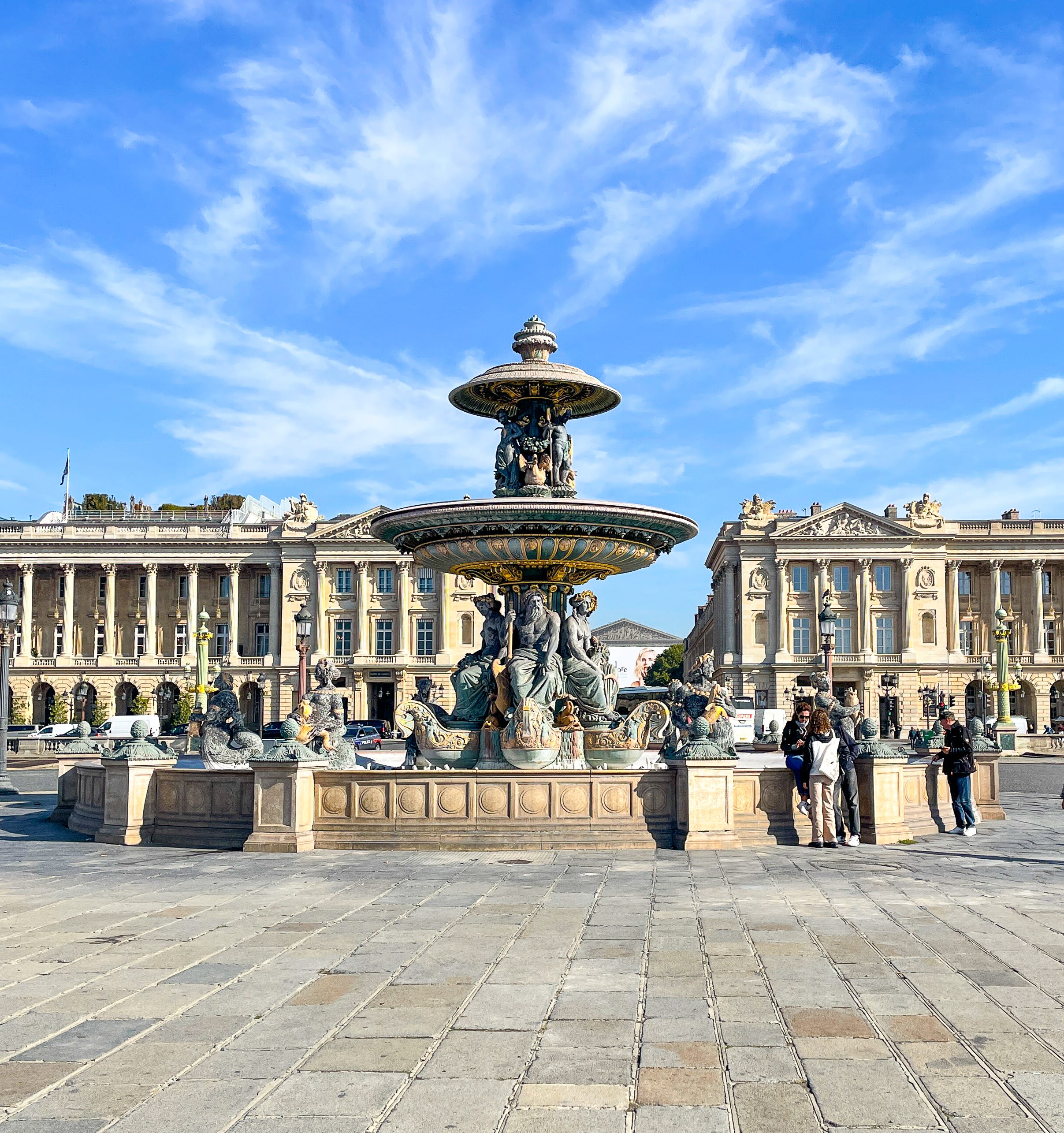This photograph captures the Fontaine de Mer in Paris, France, showcasing the intricate design and majestic beauty of this renowned European landmark. The center of attention is the ornate fountain, adorned with detailed statues of figures in robes or tunics, likely representing Greek gods. These figures are seated at the base, appearing regal as if upon thrones, and are complemented by another tier of statues and animals holding up a large, plate-like structure. The statues themselves exhibit a green hue, indicative of oxidized copper or bronze, with elements of gold ornamentation adding to their splendor. Encircling the fountain are a few onlookers, emphasizing its attraction as a popular gathering spot. Behind the fountain, large buildings with tannish brown stonework and grand columns complete the scene, set against a partly cloudy sky with streaks of white amidst the bright blue backdrop, enhancing the overall picturesque ambiance of this iconic Parisian destination.